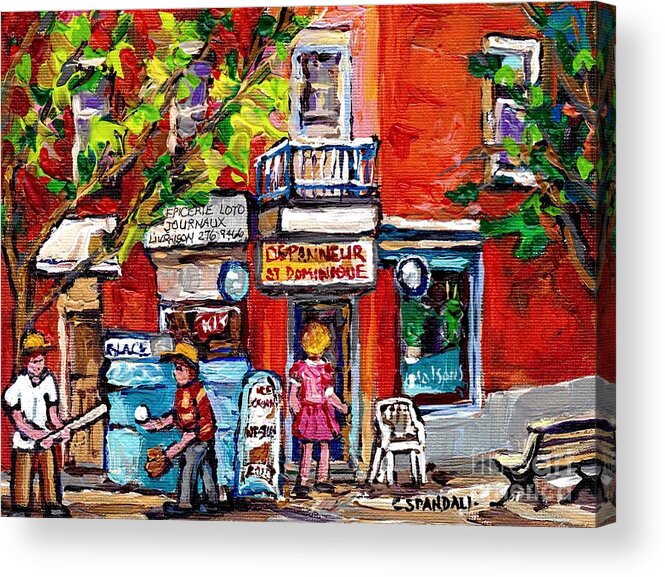The artwork appears to be an intricately detailed painting on a three-dimensional rectangular canvas, possibly depicting a quaint French or Montreal-style café located on a bustling street corner. The focal point is a red brick building which stands prominently in the center of the composition. At the entrance, a blonde woman in a pink dress is about to walk inside, under a sign that reads "Le Pontier Saint Dominique." Above her, there is a small balcony with a door and several windows—two on the left partially obscured by a tree with lush green foliage, and one on the right. 

In the foreground, on the left side, two young boys are engaged in a game of baseball. One boy, with brown hair, a yellow cap, a white shirt, and brown pants, is holding a baseball bat and faces the other boy. The second boy, wearing a yellow hat, a red and yellow shirt, and blue pants, has a ball in his left hand and a glove on his right. A blue dumpster is situated behind the second boy.

The scene is enriched with additional details: a white chair facing the viewer sits to the right of the café entrance, accompanied by a window adorned with green plants and a blue banner above it. Near the bottom right of the painting, the artist’s signature, "C. Standali," is visible. The charming and lively tableau is framed further by the presence of another street sign in French, a park bench, and a tree extending into the composition from the right side. The painting captures a vibrant street scene bathed in daylight, bustling with activity and nostalgia.